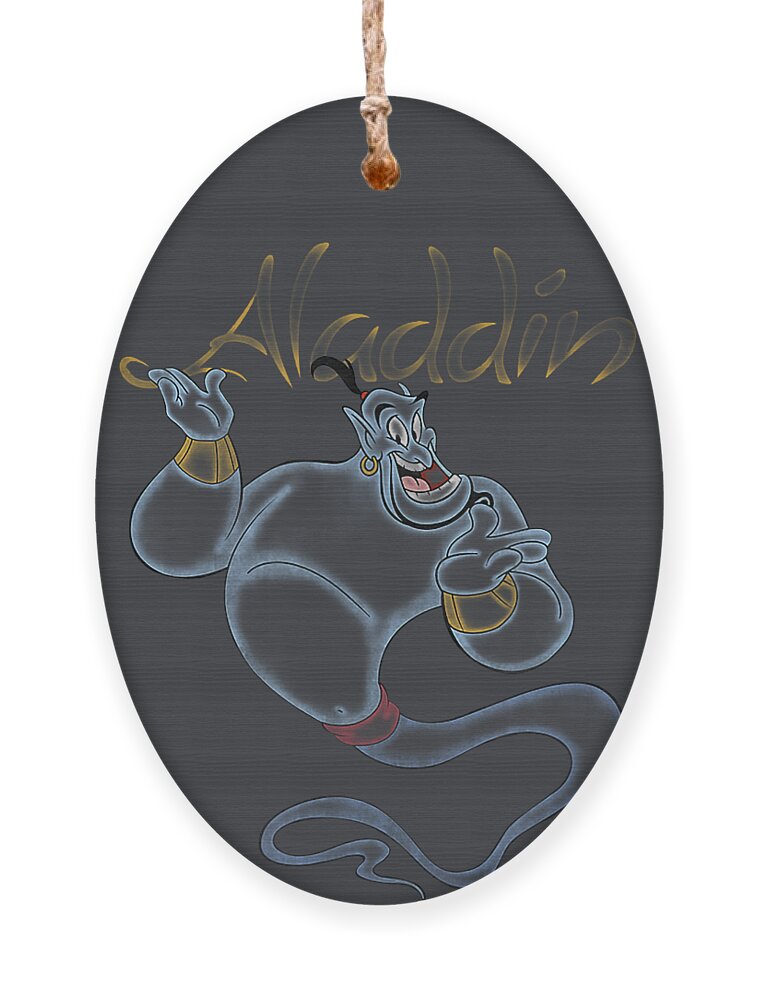This image features a close-up of an intricate Disney-themed pendant or ornament inspired by the movie "Aladdin." The pendant, which is oval and somewhat egg-shaped, is dark gray with hints of black and lighter gray hues, and it hangs from a beige, rope-like string threaded through a hole near its top. The surface of the pendant has a horizontal grain pattern.

Prominently displayed on the pendant is a depiction of the Genie, rendered in an almost neon-like outline or painting that spans from the bottom to about three-quarters of the way to the top. The Genie is vividly blue, with a wide, gaping smile, eyes looking slightly to the right, and a gold earring in one ear. His black ponytail is tied with a red band, and he sports two gold bracelets on his wrists. His arms are positioned up near his shoulders as if in the act of granting a wish. A red sash is wrapped around his midsection, and his form tapers sinuously into a wispy, spiraled tail that curves like a snake and ends in a sharp point at the bottom of the oval.

Above the Genie's figure, the name "Aladdin" is written in flowing gold letters. While some parts of the lettering appear vibrant, others seem intentionally faded, akin to a flickering neon sign, adding an additional layer of magical allure. This detailed portrayal captures the whimsical essence of the beloved character and the enchanting world of "Aladdin."